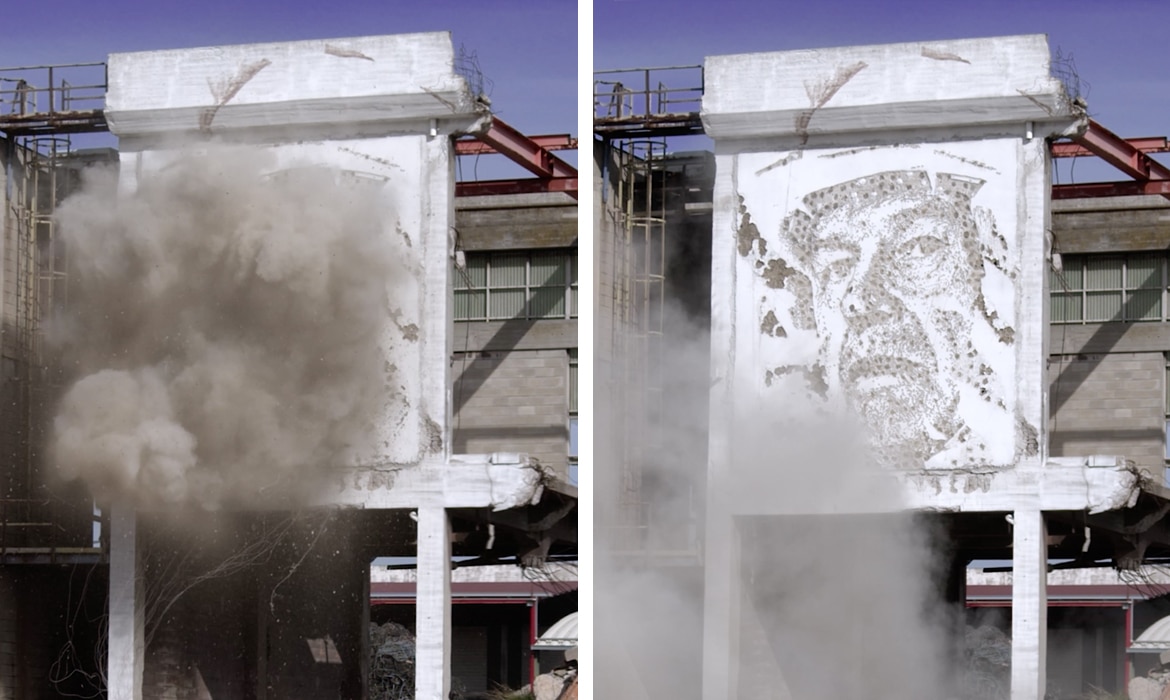This image is a composite of two photographs positioned side by side, capturing an industrial outdoor scene at different times. The left photograph shows an industrial area with a concrete building featuring red steel beams and two square columns. In the background, a factory wall is visible under a blue sky. A large plume of smoke obscures a white panel, leaving only its frame and edges discernible. The panel appears to hang from a wooden post. The right photograph reveals the same scene after the smoke has dissipated, uncovering a black and white illustration on the white panel. The illustration depicts a man's face, likely donning what appears to be a fireman's helmet, turned slightly to the side. The sequence of photos suggests a "before and after" scenario, possibly highlighting the artistic transformation of the setting through the movement of smoke, resembling art created by blasting techniques such as dynamite blasts.